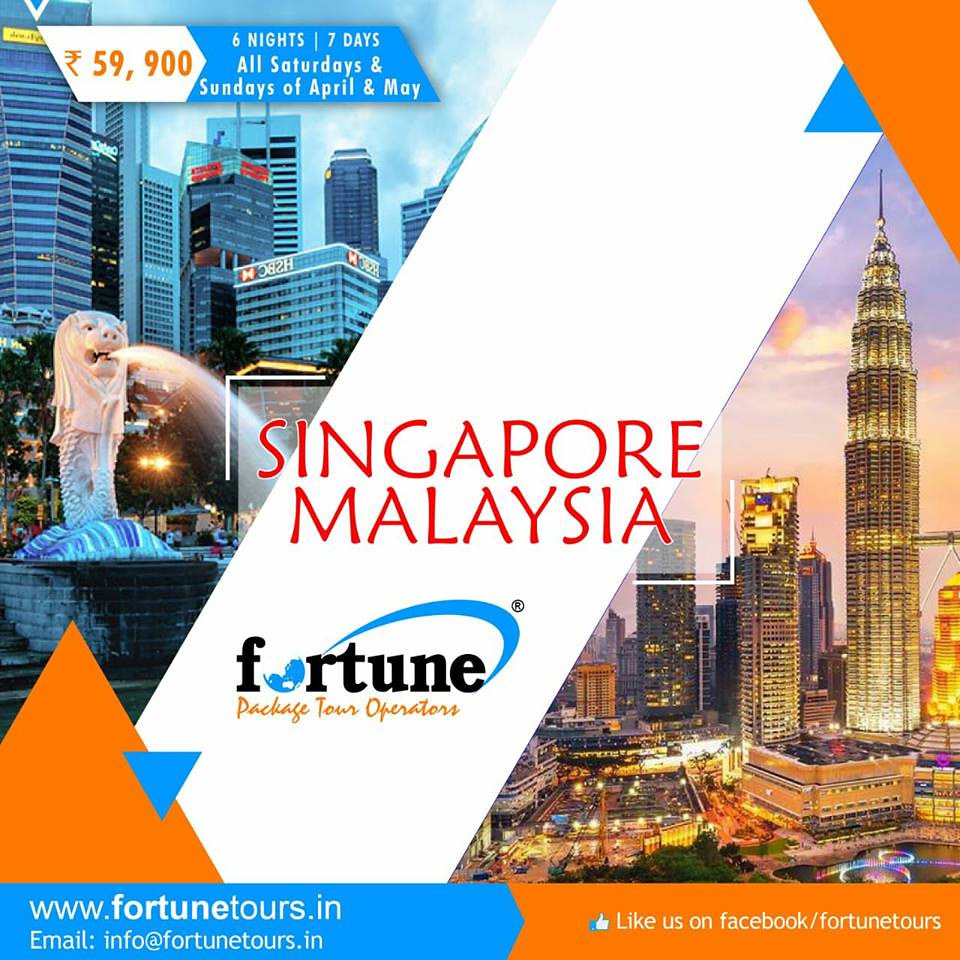The advertisement poster features a vibrant cityscape in the background, showcasing various multi-story buildings and statues, likely from Malaysia and Singapore. Among the notable elements is a statue of a lion-headed fish, serving as a fountain. An orange-colored triangle is positioned in the top right corner, adding a pop of color. Prominently displayed in the middle of the poster is the text "Singapore, Malaysia, Fortune Package Tour Operators." The top left corner lists the price "₹59,900" for a travel package that spans "6 nights, 7 days" and is available "all Saturdays and Sundays of April and May." The bottom left corner provides the website "www.fortunetours.in" and email "info@fortunetours.in" for further inquiries. On the bottom right, there is a prompt to "Like us on Facebook / Fortune Tours." The poster effectively blends images and essential details to entice prospective travelers.